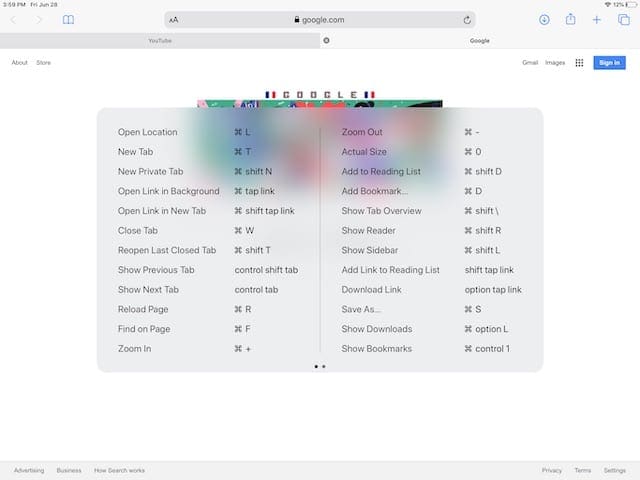Screenshot Captured on an Apple Device Featuring a List of Browser Commands

This detailed image showcases a screenshot taken on an Apple device, with the browser currently set to Google.com. The browser displays two open tabs: one for YouTube and one for Google, with the screenshot specifically focusing on the Google tab.

The image provides a comprehensive list of browser commands split into two distinct columns. Here is an exhaustive breakdown of these commands:

**Left Column:**
- **Open Location:** Command (⌘) + L
- **New Tab:** Command (⌘) + T
- **New Private Tab:** Command (⌘) + Shift (⇧) + N
- **Open Link in Background:** Command (⌘) + Tap Link
- **Open Link in New Tab:** Command (⌘) + Shift (⇧) + Tap Link
- **Close Tab:** Command (⌘) + W
- **Reopen Last Closed Tab:** Command (⌘) + Shift (⇧) + T
- **Show Previous Tab:** Control (⌃) + Shift (⇧) + Tab
- **Show Next Tab:** Control (⌃) + Tab
- **Reload Page:** Command (⌘) + R
- **Find On Page:** Command (⌘) + F
- **Zoom In:** Command (⌘) + "+"
  
**Right Column:**
- **Zoom Out:** Command (⌘) + "-"
- **Actual Size:** Command (⌘) + "0"
- **Add to Reading List:** Command (⌘) + Shift (⇧) + D
- **Add Bookmark:** Command (⌘) + D
- **Show Tab Overview:** Command (⌘) + Shift (⇧) + Backslash (\\)
- **Show Reader:** Command (⌘) + Shift (⇧) + R
- **Show Sidebar:** Command (⌘) + Shift (⇧) + L
- **Add Link to Reading List:** Shift (⇧) + Tap Link
- **Download Link:** Option (⌥) + Tap Link
- **Save As:** Command (⌘) + S
- **Show Downloads:** Command (⌘) + Option (⌥) + L
- **Show Bookmarks:** Command (⌘) + Control (⌃) + 1

This organized list of keyboard shortcuts is a handy reference for efficient browsing and navigation on Apple devices.